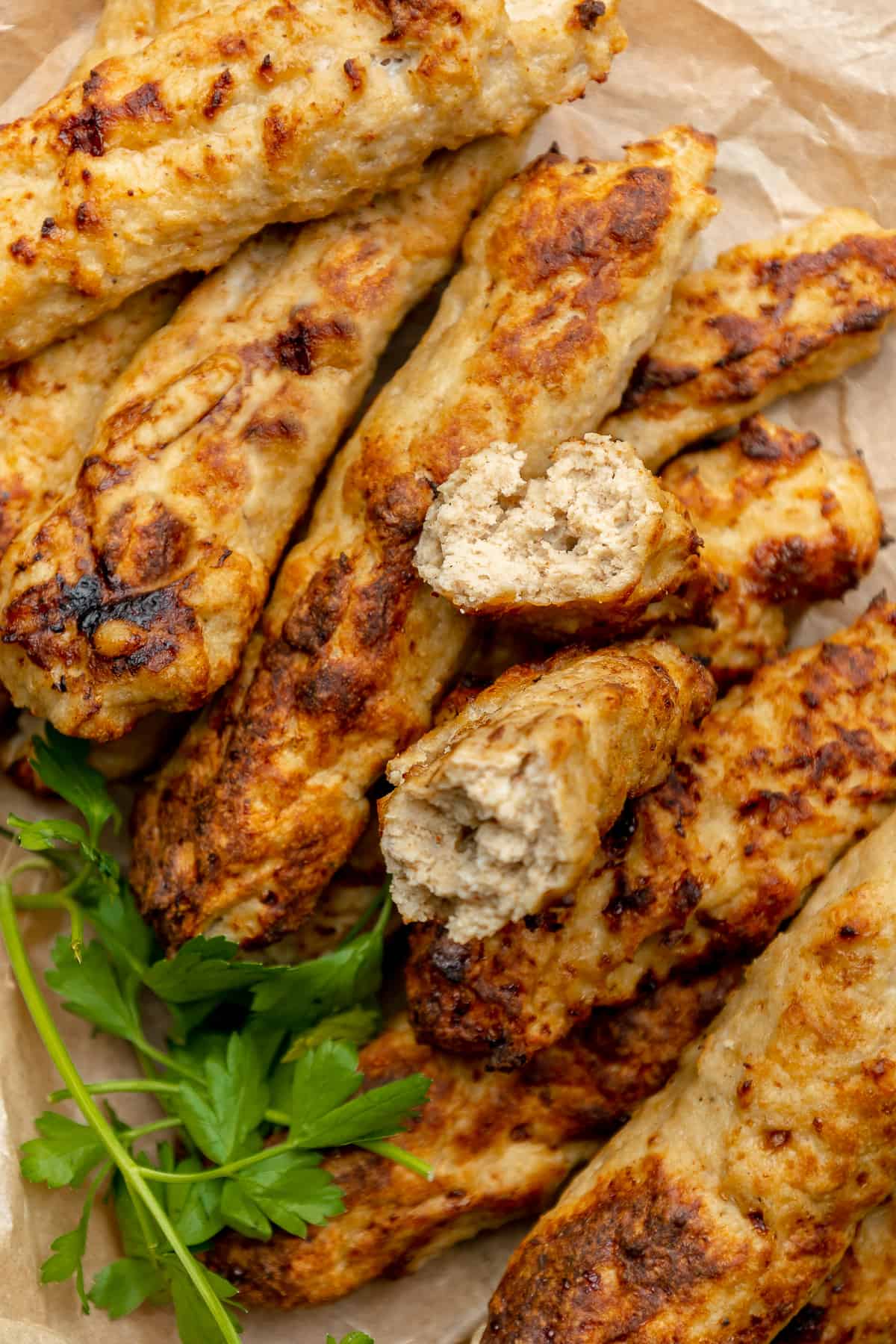The image showcases a variety of golden-brown, finger-shaped snacks, resembling breadsticks or possibly fried pastries, arranged on a crumpled sheet of brown parchment paper. The center of the composition features one of these snacks broken in half, revealing a light, creamish-brown, crumbly interior. The snacks are evenly browned, with slight crisping and darker patches suggesting they have been baked or fried. In the bottom left corner, there is a delicate sprig of cilantro adding a touch of green to the arrangement. The parchment paper beneath displays visible crinkles and a semi-transparent texture, particularly noticeable in the top right and bottom left areas of the image.